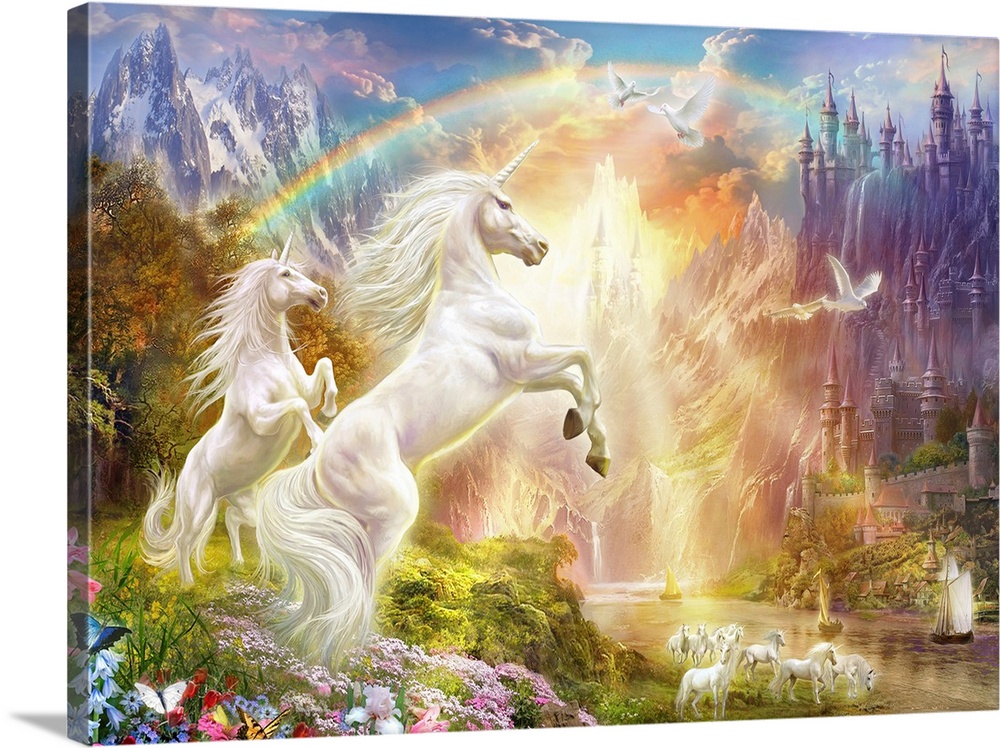This detailed painting on a square canvas vividly depicts a vibrant fantasy world. The central focus is on two majestic white unicorns, rearing up as if galloping or neighing towards a brilliant rainbow arching above them. Their flowing white manes and fluffy tails catch the rays of intricate sunlight filtering through the scene. Directly below, more unicorns graze and drink from a serene river coursing through a lush, grassy landscape dotted with various colored flowers—blue, pink, and red—and adorned with trees exhibiting a spectrum of green, red, and brown leaves. 

To the right of the unicorns, perched on a purple cliff, stands an imposing castle with grand beige walls and towering purple spires, accompanied by more spires below it. The castle's fantasy architecture enhances the whimsical aura of the scene. The left side showcases a mountain range accented with snowy patches, complementing the greenery below. 

In the sky, beyond the rainbow's blue, red, and yellow hues, a white bird soars, symbolizing freedom and harmony. Another white bird is seen gliding along the river, further adding to the idyllic setting. The entire composition, filled with every imaginable color, exudes a joyful and enchanting atmosphere, bringing to life a mesmerizing medieval fantasy landscape designed to captivate and delight.